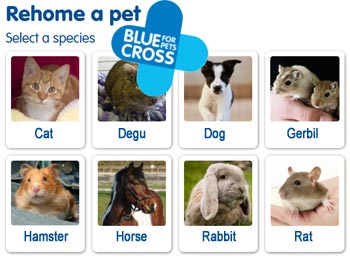The image features a collage of four distinct pictures, each showcasing a different animal species, accompanied by respective labels. The backdrop of the collage presents the text "Re-home a Pet" and "Select a Species," hinting at an adoption platform. The "Blue Cross for Pets" logo is prominently displayed, suggesting the organization behind the initiative. 

1. The first section depicts a picture of a cat with the word "Cat" beneath it.
2. The second section shows an image supposed to represent a "Degoo," though the logo partially obscures this particular animal, making it hard to identify.
3. The third section includes a photograph of a black or brown dog with the label "Dog."
4. The fourth section displays two gerbils being held, underlined by the word "Gerbil."
5. Other sections in the collage include:
   - A solitary hamster pictured with the label "Hamster."
   - A majestic horse image with the caption "Horse."
   - A grey rabbit with the designation "Rabbit."
   - Lastly, a rat held in someone's hand, succinctly titled "Rat." 

The collage visually promotes the diversity of pets available for adoption through the Blue Cross for Pets re-homing service, spanning across eight categories, including cats, degus, dogs, gerbils, hamsters, horses, rabbits, and rats.